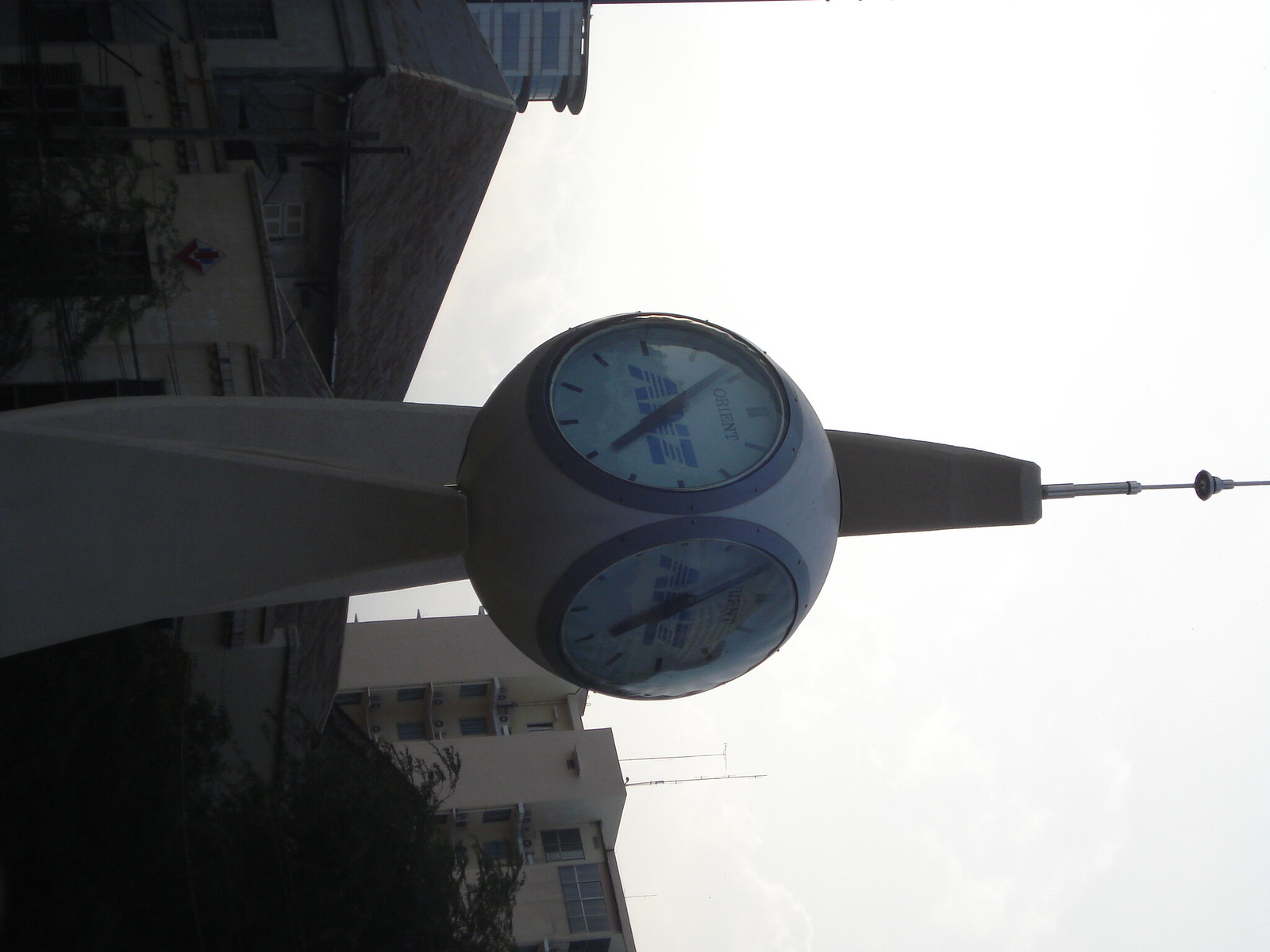This outdoor image features a unique, futuristic-looking clock turned on its side. Mounted on a stone base that tapers upward to a spherical stand, the clock itself resembles an astronaut helmet, with multiple clock faces positioned around its rounded surface. Although presented horizontally, the clock’s spire, originally at the top, points to the right. Displaying Roman numerals and black clock hands on its white face, the clock reads six minutes to five. Around the middle, there are blue letters outlined in white, possibly spelling "A-N-Z". The clock's brand "Orient" is also visible. The background includes several beige-colored, multi-story buildings and some trees, enhancing the outdoor setting.